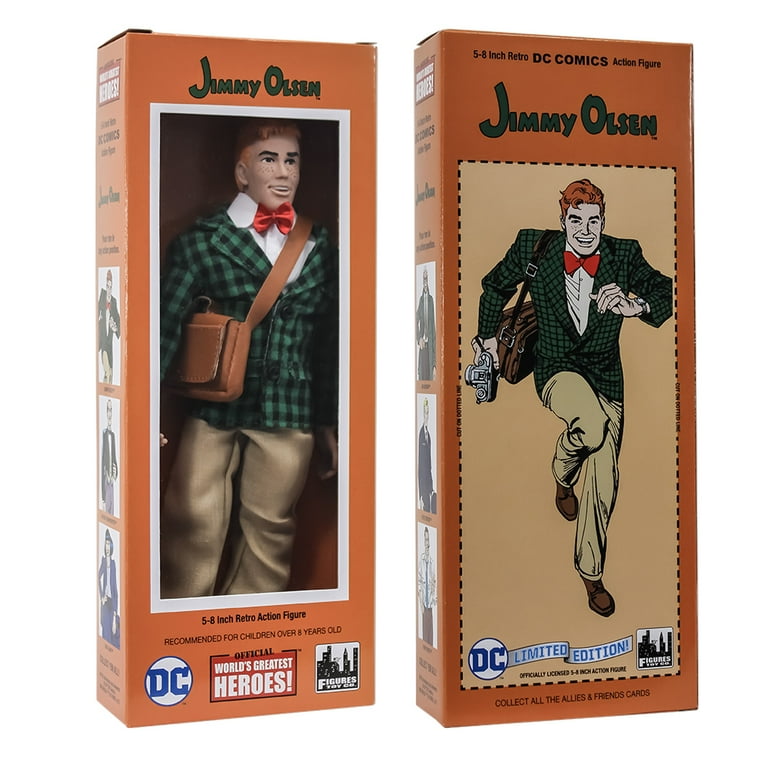This image features a detailed view of a Jimmy Olsen retro action figure. The figure is housed in a dull orange box with a clear cutout window that showcases the doll inside. The top of the box prominently displays the name "Jimmy Olsen" in black text. The doll is designed as a boy with freckles, reddish hair, and is smiling with black eyebrows. He is dressed in a distinct outfit comprising a red bow tie, white shirt, green and black checkered jacket, and khaki pants. Additionally, he carries a brown over-the-shoulder bag on his left side. Beneath the window, the box indicates that this is a 5 to 8-inch retro action figure recommended for children over 8 years old.

On the left side of the front of the box, there's a DC logo, and on the right, another logo noting "Official World’s Greatest Heroes." The back of the box features a drawing of Jimmy Olsen in motion, presumably running, alongside the same color scheme and branding elements. Text at the bottom of the back side includes "DC limited edition figures" and promotes the collection of "all allies and friends cards."